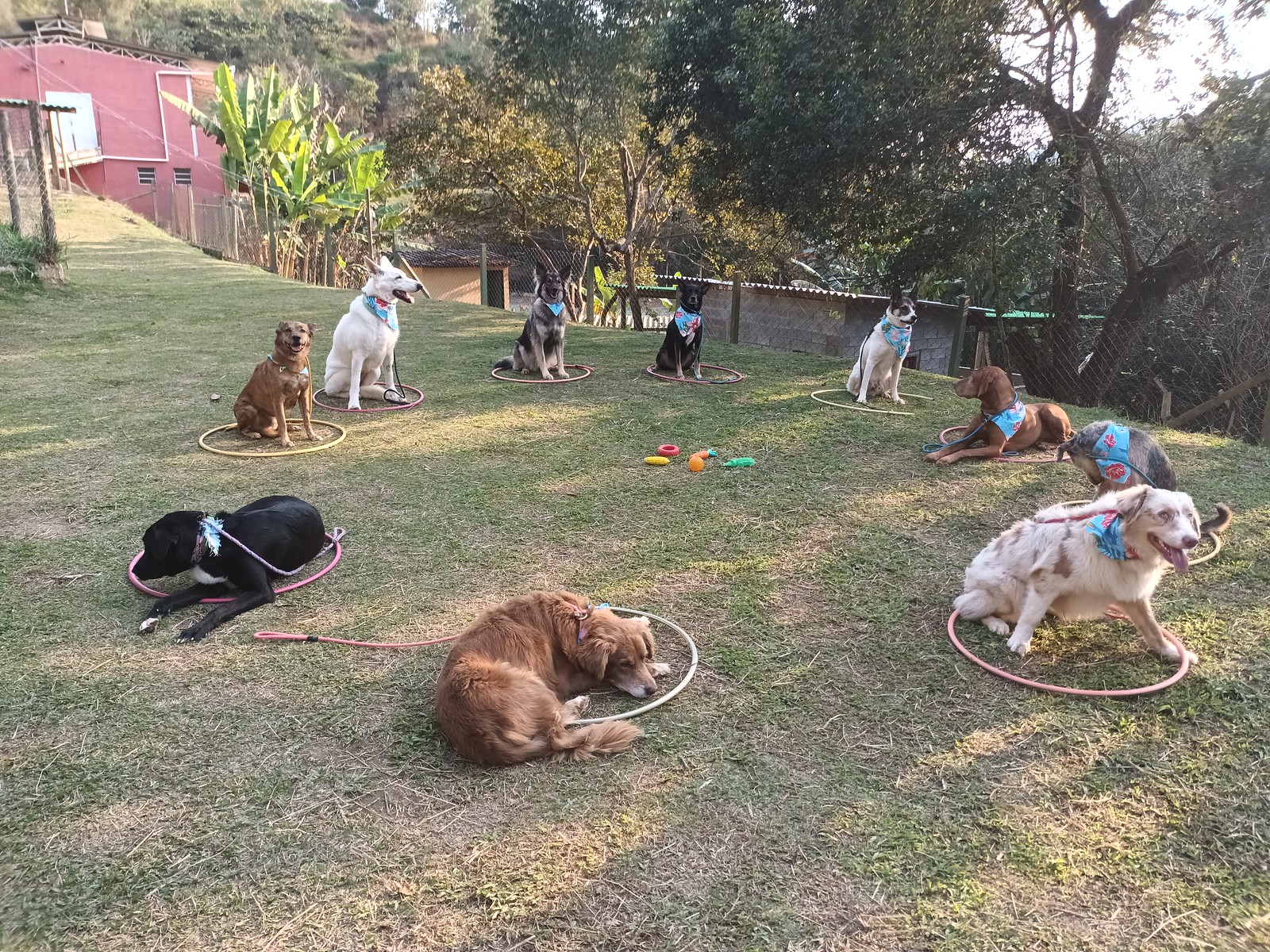In the image, a group of ten diverse dogs are each positioned within a hula hoop, forming a circular arrangement on a hill with short grass. Each hula hoop encircles the dogs, which vary in breed, size, and appearance. Notably, a large white dog with brown patches sits in the foreground, while a brown dog in a side view position lies within its hoop. A German Shepherd mix with light brown and black fur, a black dog with a light blue bandana, and a white dog with black ears and face are among the dogs present. The dogs are all either sitting or lying in their respective hoops, with various toys or objects placed in the center. In the background, a red house stands surrounded by green foliage and diverse trees. Additionally, a cinder block structure is visible in the middle of the photo, enhancing the tranquil, photogenic scenery.